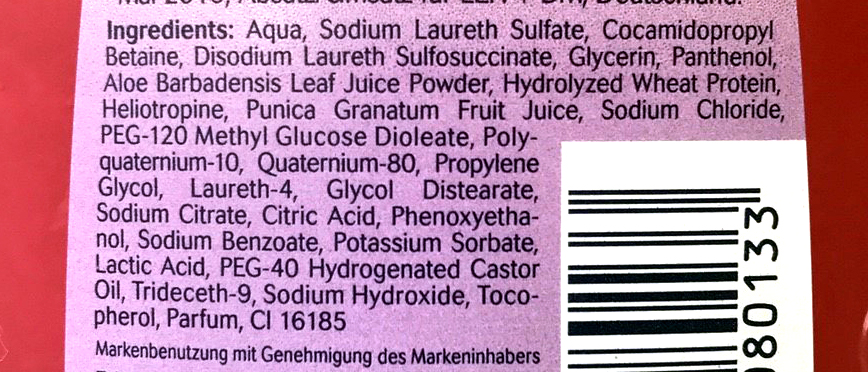This close-up image captures the label of a hair care or skin care product bottle. The label itself features a soft pinkish-purple background with black text, providing a striking contrast for easy readability. The bottle design includes red accents visible on either side of the label. The bottom right corner of the label is occupied by a white barcode with black stripes, essential for retail scanning. Below a lengthy list of ingredients, there is a section of text that appears to be in German, adding an international touch. The ingredients list is detailed and extensive, starting with aqua (water), sodium laureth sulfate, cocamidopropyl betaine, disodium laureth sulfosuccinate, glycerin, panthenol, and aloe barbadensis leaf juice powder, among others.